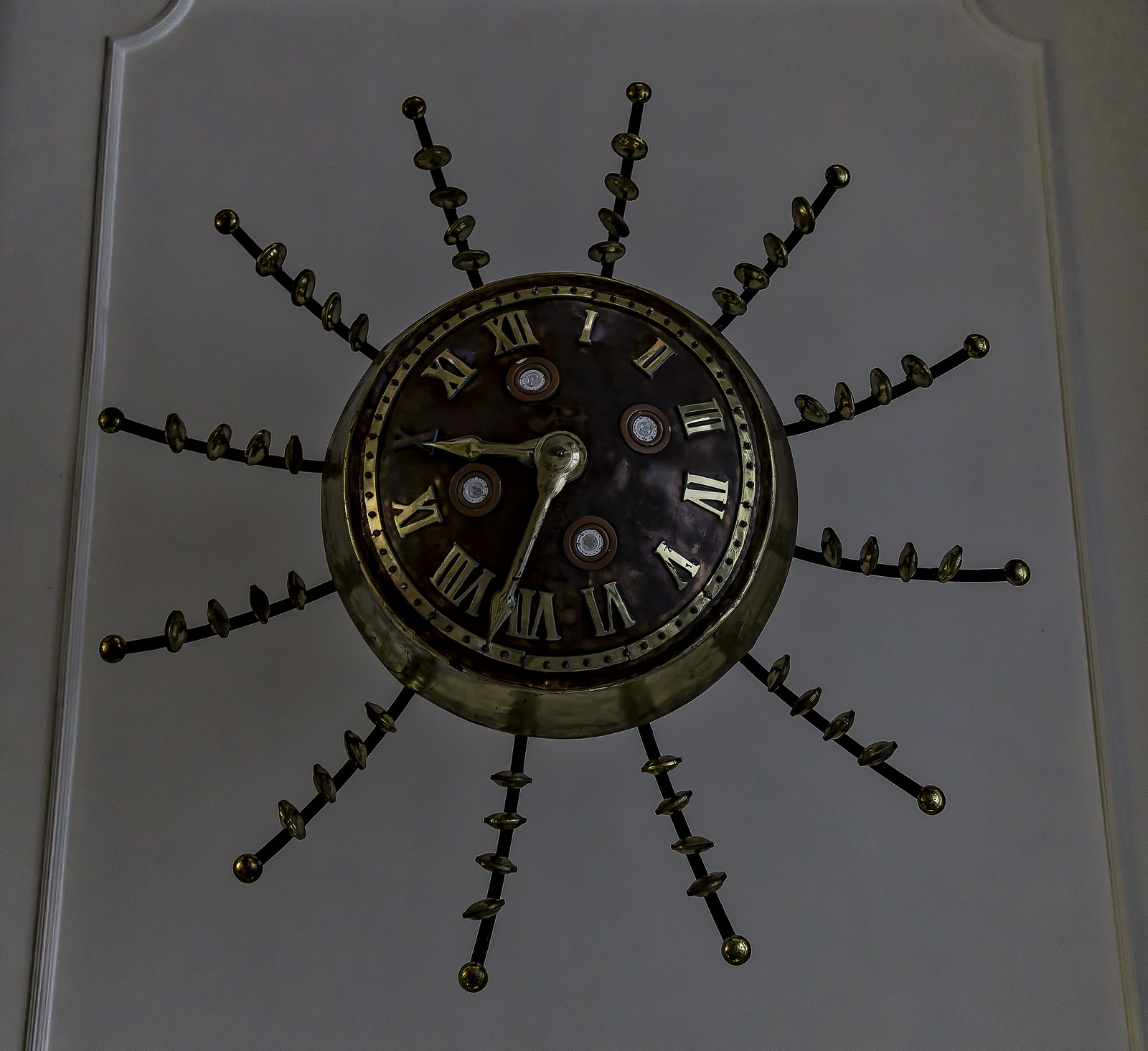This image features a stylish wall-mounted clock with an intricate design. The clock itself is predominantly black with an elegant brass outline. The face of the clock showcases Roman numerals in a shimmering gold or brass color, adding a touch of classic sophistication. According to the clock, the time is approximately 9:35 or 9:36.

The clock is mounted within a larger frame that is partially visible, further enhancing its decorative appeal. Extending from the clock are 12 spokes, one corresponding to each Roman numeral hour marker. Each spoke is meticulously adorned with four small circles spaced evenly along its length, culminating in a small ball at the very end. This detailed and ornate design adds a unique and decorative flair to the clock, making it not just a timepiece, but a statement piece of decor.